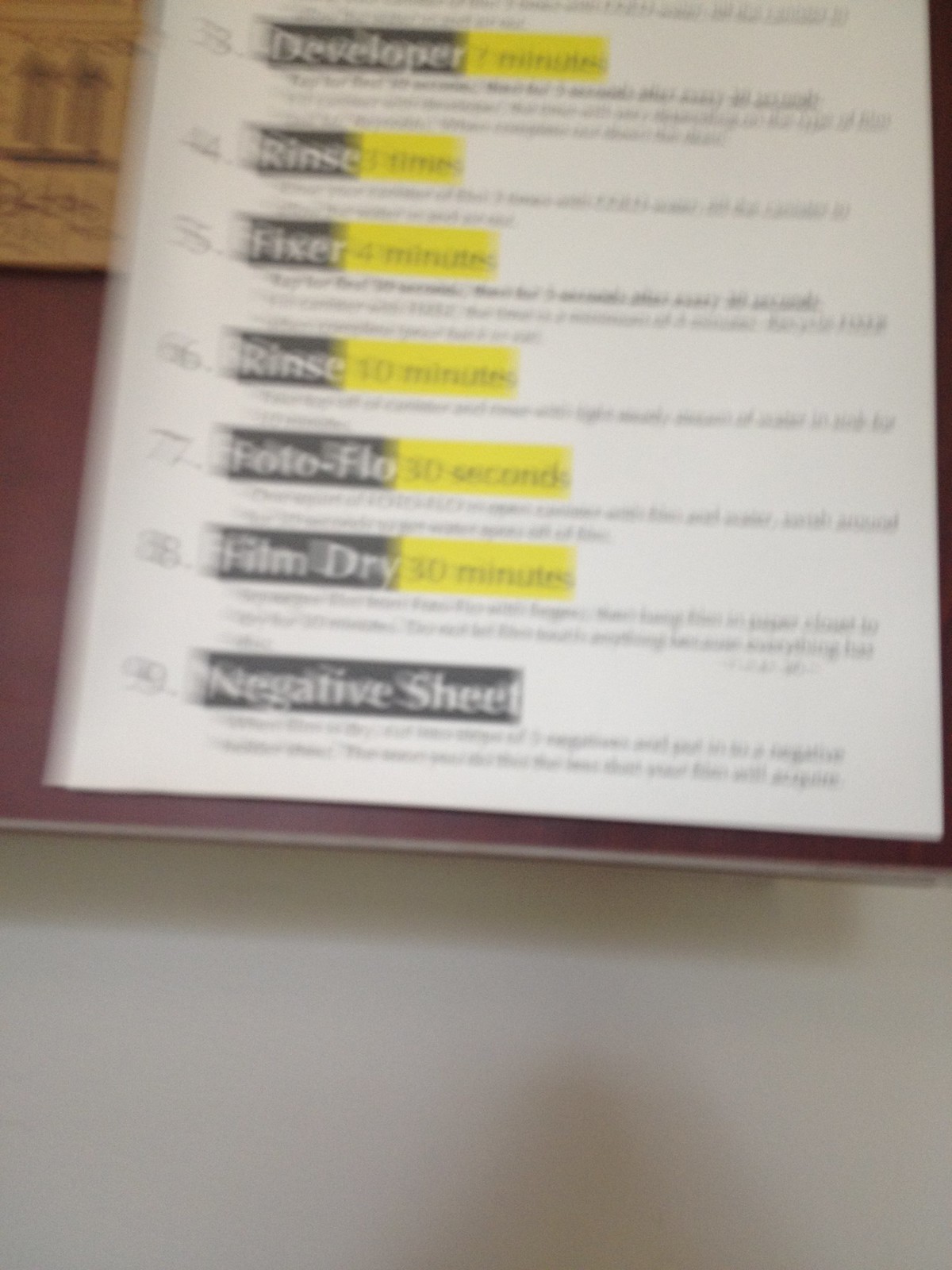This image captures a very blurry close-up photograph of an instructional sheet for film developing, likely taken vertically from a first-person perspective on a phone. The white sheet of paper, partially visible, depicts steps 3 through 9 of a film development process, and is positioned on a white table. The top part of the sheet, steps 1 and 2, are cut off in the view. Bolded categories beside numbered steps are faintly discernible, and the sheet seems to have black text with yellow highlighted timings.

Step 3 appears to be "Developer" with a yellow box next to it indicating "7 minutes," followed by a paragraph of instructions that are too blurred to read. Step 4 says "Rinse," but the exact time is indiscernible due to the blur, alongside a yellow box and more illegible text. Step 5 reads "Fixer, 4 minutes." Step 6 mentions "Rinse" again, with a time that remains unclear. Step 7 lists "Photo Flow," possibly written as "FOTO-FLO," but the time is not readable. Step 8 is "Film dry," again with an unclear duration. Finally, step 9 states "Negative sheet."

The instructional sheet seems to be resting on a piece of cardboard in the top left corner and a maroon-colored notebook beneath it. This overall composition suggests a practical workspace setting for film developing.